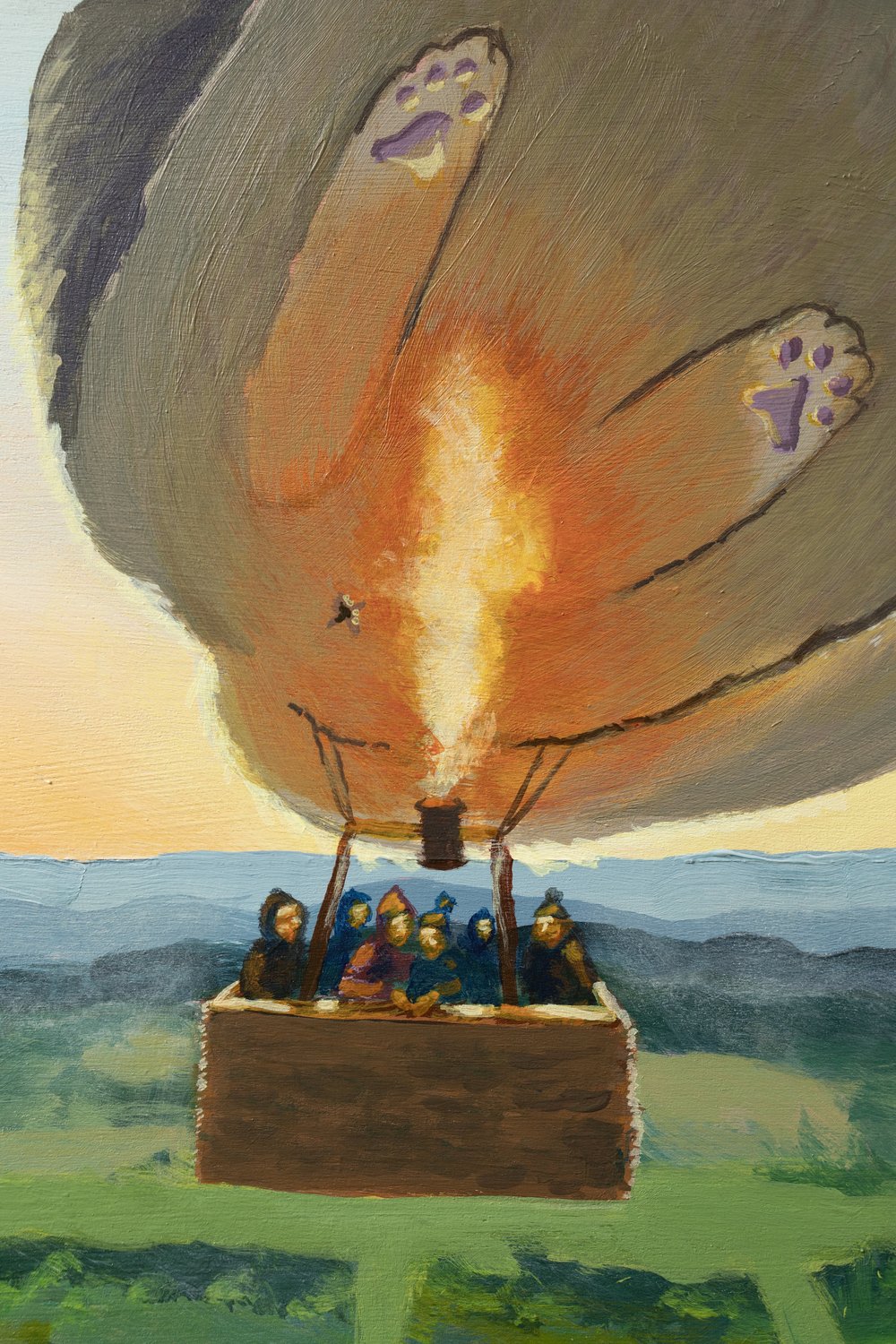The image is a whimsical watercolor painting featuring a hot air balloon with an unconventional twist. Instead of a traditional balloon, a large grayish cat's hind legs and tail take its place, with a distinctive cat butthole marking in the center, forming an X. The fire that propels the balloon appears to be fueled humorously by the cat, adding a playful element to the scene. The square wooden basket attached below houses six indistinctly detailed people. They are floating high above grassy fields, which are subtly depicted in shades of green, bathed in the warm hues of an orange and blue sunset sky. The entire scene captures a blend of surrealism and whimsy, creating an imaginative and eye-catching spectacle.